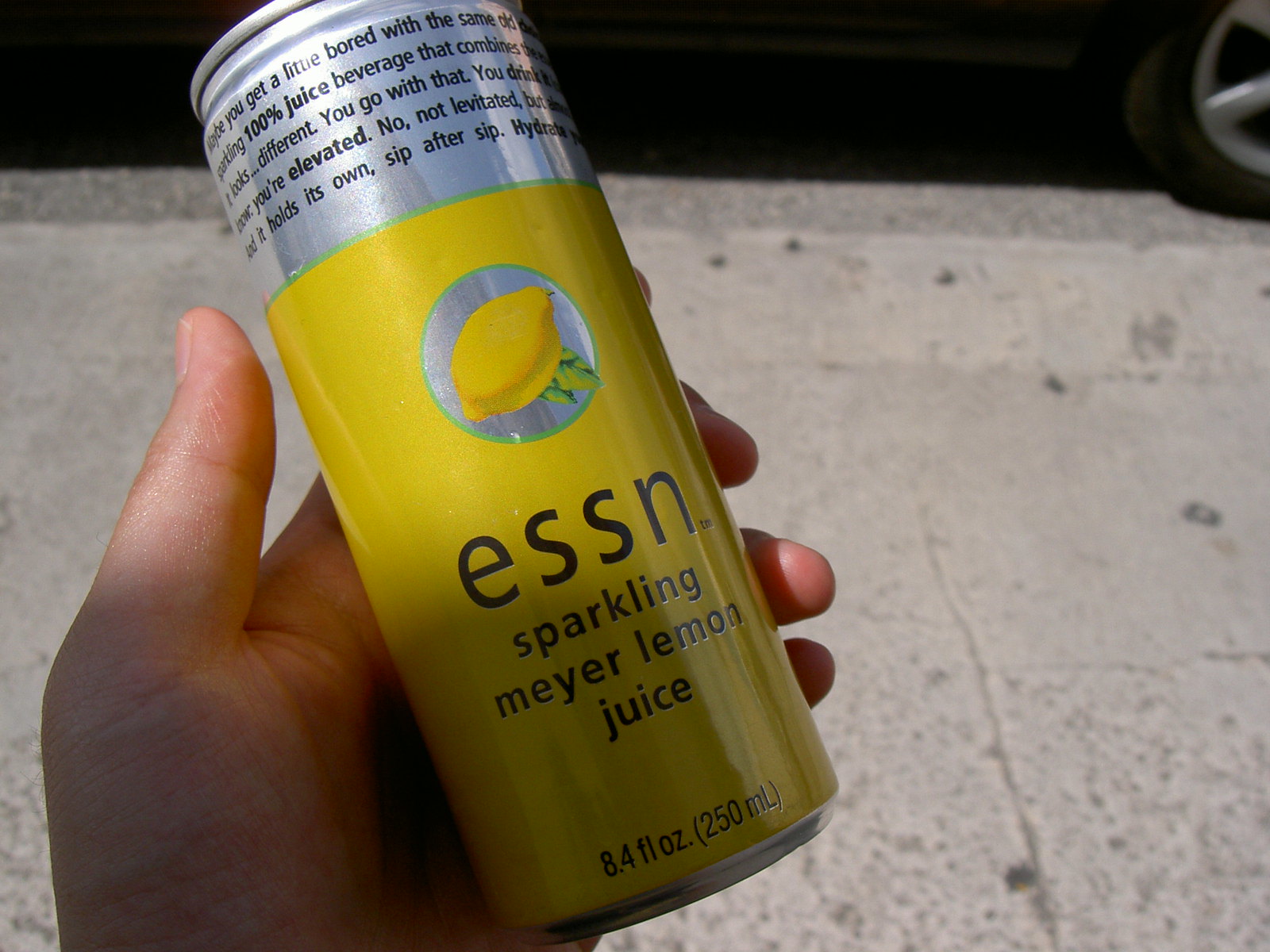The image is a close-up photograph focusing on a person's left hand holding a slender aluminum can. The can is distinctly shown with a yellow bottom section and a silver top section. The can features various design elements: prominently, there's the text "ESSN" in black on the yellow portion, followed by "Sparkling Meyer Lemon Juice" in smaller black text beneath it. At the bottom, it clearly states "8.4 fluid ounces (250 milliliters)." A circular silver detail also appears on the yellow section, containing a bright yellow lemon with green leaves. The top third of the can is silver with additional text that is partly legible and describes something about the beverage. The hand holding the can is partially shadowed near the bottom, with sunlight illuminating the area near the thumb and above. The background shows a concrete gray sidewalk with a car tire and hubcap visible in the top right corner, as well as some shadowing beneath the car.